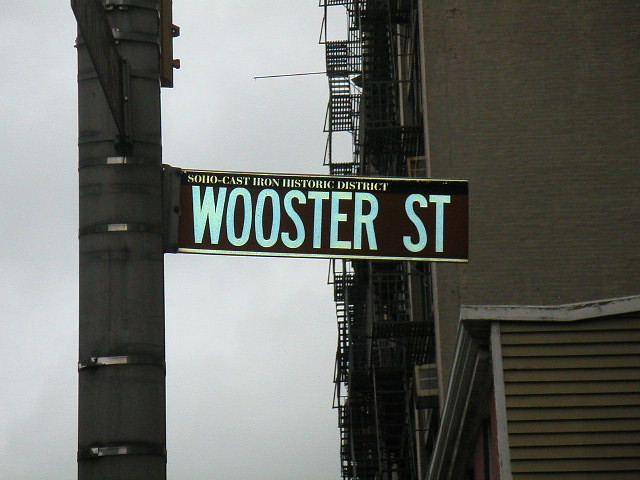The photograph, taken outside under a gray, cloudy sky tinged with pale lilac, prominently features a metal pole on the left side. The pole holds a street sign that captures the viewer's attention, reading "Soho Cast Iron Historic District" and "Worcester Street" in white lettering against a brown rectangular background with a black border. The pole is a grayish-brown color, blending slightly with the overcast sky. To the right of the pole is a cinder block building with a metal fire escape running down its facade, adding texture and an urban feel. In the lower right corner, part of another building with brown vinyl siding and some metal roofing is visible. This urban scene hints at a bustling, downtown area characterized by historic districts and architectural details.